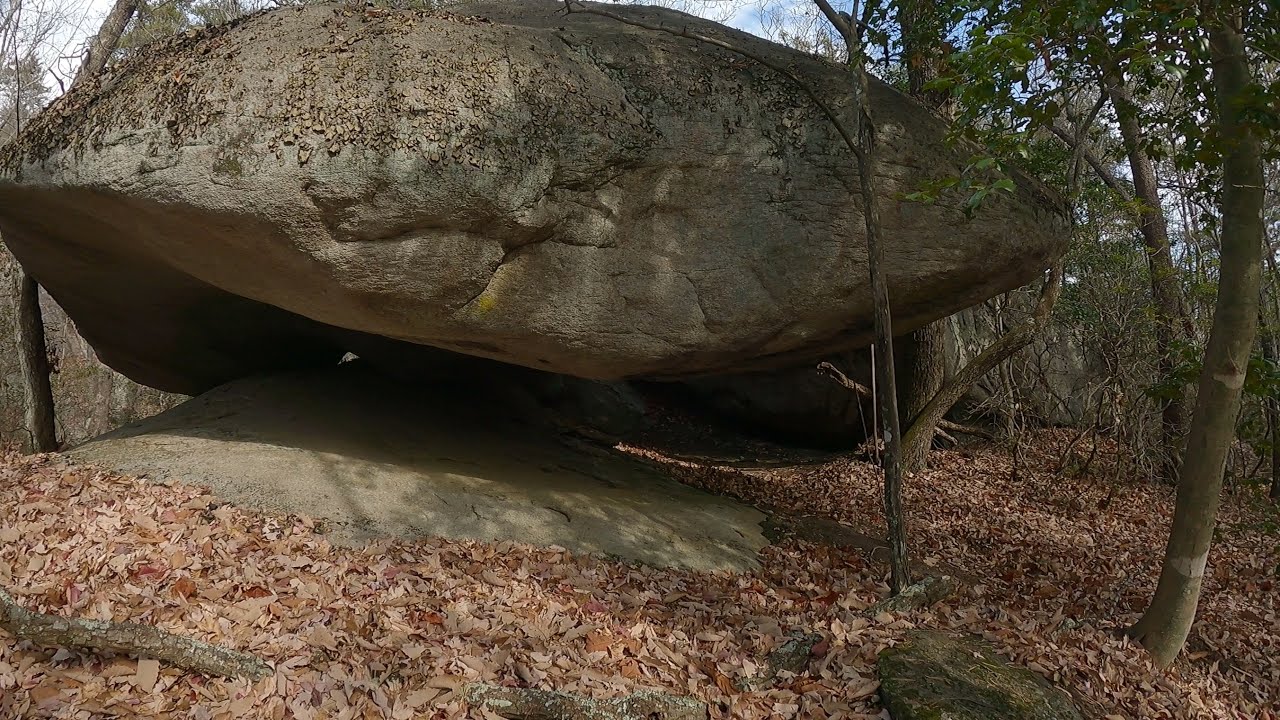In a serene forest bathed in autumn light, the focal point of the image is a large, monolithic gray granite boulder that appears to be hovering slightly above the ground. This rounded, smooth-edged boulder is precariously balanced on another rock outcropping, creating a sheltered, shadowy nook underneath. The forest floor is blanketed in a dense layer of rusty, reddish-brown fallen leaves, interspersed with occasional rock fragments peeking through. The scene is framed by numerous trees, with some displaying green foliage to the right, while others in the distance stand bare. Sunlight filters through the canopy, casting shadows on the right half of the boulder and illuminating the varied textures and colors of this tranquil woodland landscape. A sliver of blue sky is visible in the background, adding to the scene's peaceful ambiance.